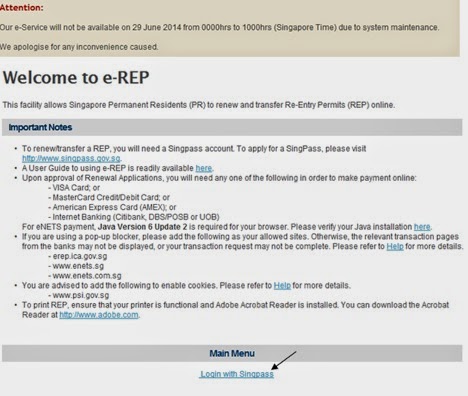The image features a website homepage with a gray-blue background. The prominent text in black font reads "Welcome to E-Rep," where the 'E' is lowercase and 'REP' is in uppercase letters. At the very top, there's a red attention box within a gray border, displaying a notice in bold red letters that reads "Attention." The notice below states: "Our service will not be available on 29 June 2014 from 00:00 to 10:00 Singapore time due to system maintenance. We apologize for any inconvenience caused."

Beneath this, the main section of the website welcomes users to E-Rep and provides a description of the service: "This facility allows Singapore's permanent residents to renew or transfer re-entry permits online." It explains that the site assists individuals who have been outside the country and wish to re-enter Singapore.

Further down, there is another gray box spanning the width of the website, featuring the heading "Important Notes" in blue font. This section contains an extensive list of important information, including contact websites and details about various types of identification that can be used for the service.